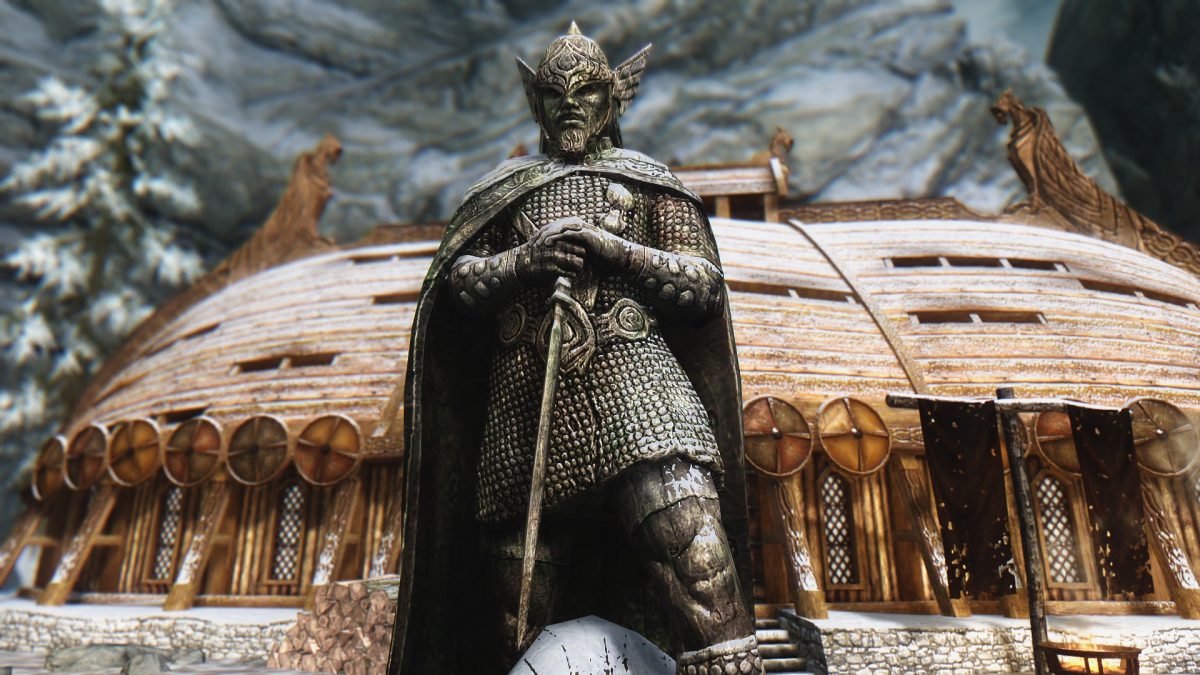In the image, a formidable statue of a warrior stands prominently in the foreground, reminiscent of a Viking or a Roman fighter from ancient times. The warrior, resembling the superhero Thor, is dressed in detailed chainmail armor and a flowing cape. His powerful stance is highlighted by the sword he grasps with both hands, planted firmly into the ground. Atop his head sits a striking helmet adorned with wings on each side, further enhancing his heroic appearance. His face is depicted with a mighty beard, suggesting a mix of Viking and possibly Asian samurai influences.

Surrounding the statue is a picturesque, snow-covered mountainous backdrop. To the left, a snowy tree blends seamlessly into the landscape. The structure behind the warrior appears to be a wooden Viking or Nordic-style hall, characterized by shields lining the border where the roof meets the building's walls. This hall, perhaps a feast hall, adds to the rich cultural ambiance of the scene. The rounded design of the building, reminiscent of an upside-down boat, and the presence of giant statues on its roof, evoke both ancient and indigenous architectural styles, further emphasizing the historical and epic nature of the setting. The entire scene is imbued with a metallic luster, giving it an otherworldly, almost futuristic quality.